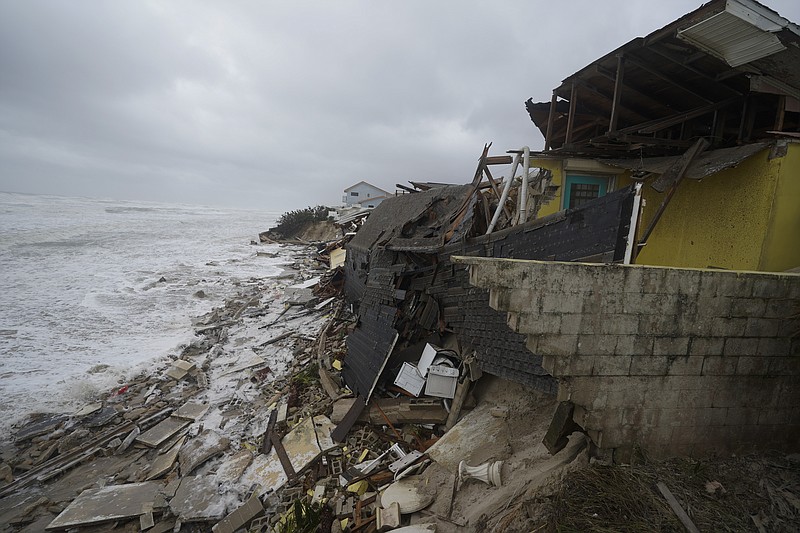The photograph captures a devastating scene of destruction along the beachfront, likely caused by a hurricane. In the foreground, various debris including cement blocks, dirt, and twigs are scattered chaotically. The central area features broken household items, with a stove partially visible amongst the rubble. To the right, the main house—with its distinctive yellow walls and an aqua-blue door—lies in ruins. Its roof has collapsed, spilling over into the sandy beach where relentless waves threaten to devour the wreckage. A shattered seawall stands as a grim testament to the storm's power. The entire landscape is painted with various shades of gray, echoing the somber mood of the overcast sky that stretches from the top left to the top right of the image. The ocean appears tumultuous, mirroring the destructive force that has laid waste to these coastal houses. Only one house in the distance seems to have escaped the widespread devastation, providing a stark contrast to the surrounding wreckage. This scene is a poignant reminder of nature's relentless fury and the fragile impermanence of human structures.